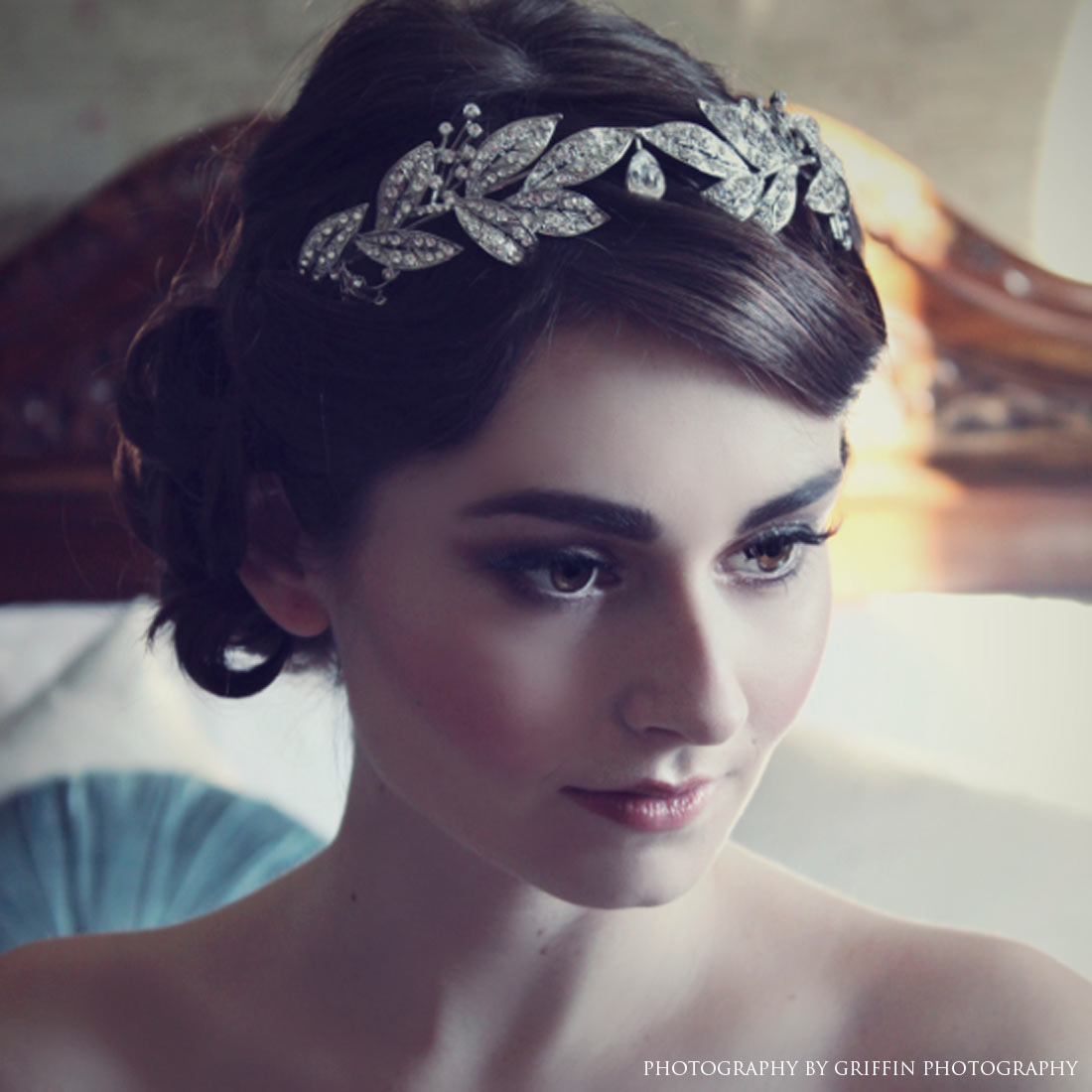This rectangular, vertically-oriented photograph, taken by Griffin Photography, features a close-up portrait of a beautiful woman. Positioned at the bottom of the frame, the woman gazes downwards and to her bottom right, exuding an air of serene contemplation. Her dark, well-defined eyebrows and carefully applied makeup, including lipstick, enhance her striking features. Her hair is elegantly styled into an intricate bun secured with a headband adorned with silver-leaf details, adding a touch of sophistication. The composition captures her from the shoulder line upwards, and the background subtly reveals a bed with a brown headboard, which frames her radiant complexion.